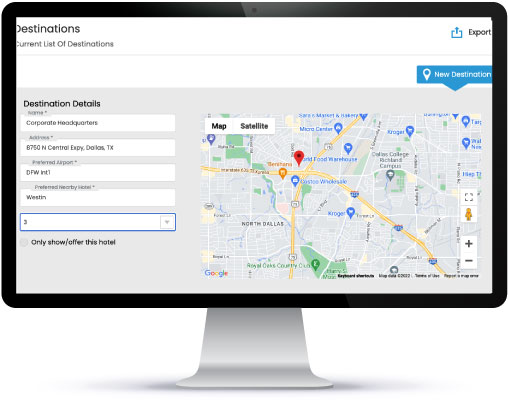The image depicts a computer-generated flat-screen monitor, standing on a small pedestal. The monitor displays a user interface for planning a trip. In the upper left corner of the screen, the label "Destination" is prominent. Below this, there is a section titled "Current List of Destinations."

On the right side of the screen, an "Export" option is available, accompanied by an export symbol. A detailed map occupies the right half of the monitor, with "Map" and "Satellite" tabs in the upper left corner of the map interface.

The left side of the screen provides detailed information about a specific destination. It includes fields for:
- **Name**: "Corporation Headquarters"
- **Address**: "8750 North Central EXPY, Dallas, Texas"
- **ZIP Code**: (this field is partially obscured or unclear)
- **Preferred Airport**: "DFW International"
- **Preferred Hotel**: The specifics are partially visible but indicate a preference for a certain hotel.

Below these details is a section with a dropdown menu, highlighted in blue. The dropdown menu has three options visible, though the exact content is unspecified. There is also a checkbox labeled “Only show/offer this hotel,” which is not selected.

The interface also includes a "New Destination" button on the right, near the top corner of the screen. The map section shows a popup in the upper right corner, which might be for additional map options or interactions.

Overall, the image represents a sophisticated, albeit virtual, trip planning software with a comprehensive interface for selecting and exporting travel destinations.